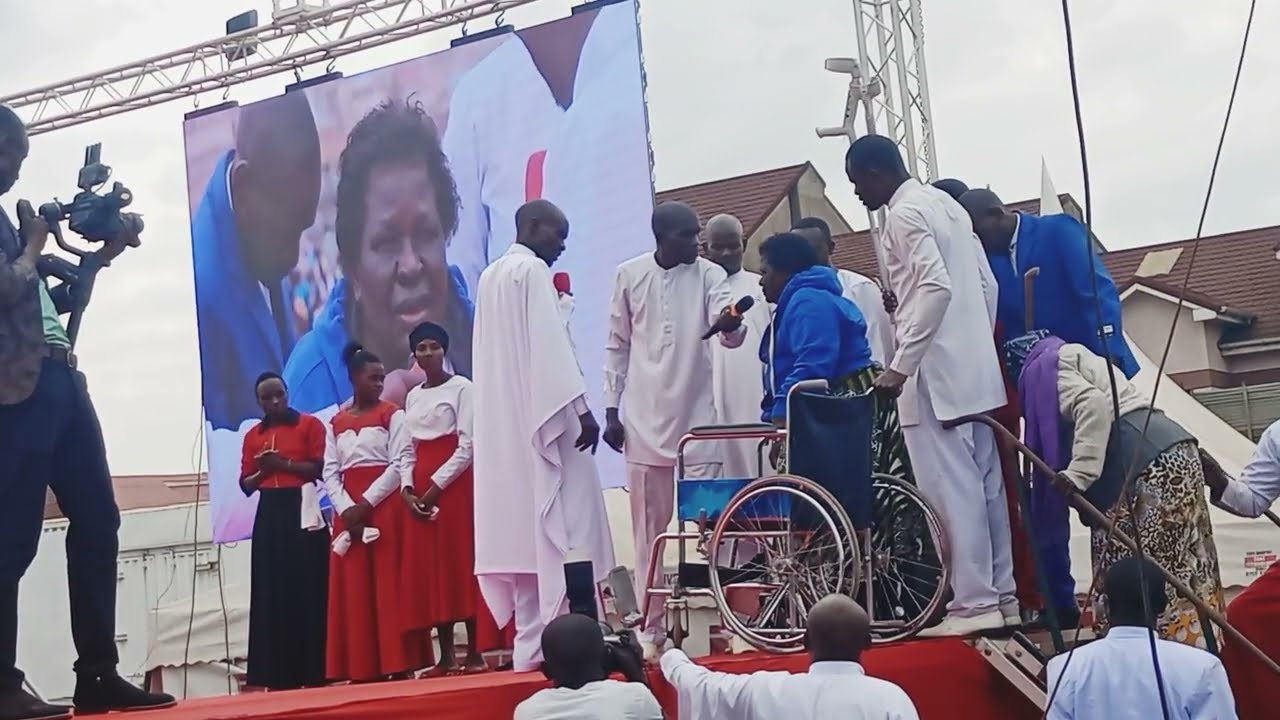The image captures an outdoor ceremony on a stage with a red floor, conveying a profound, possibly religious spectacle. Dominating the scene are three women in elegant long dresses—the one on the left in a black dress, and the other two in red dresses with accompanying white tops. The backdrop features a large screen displaying a framed picture of a woman, creating a focal point that ties the on-stage activities to the audience. Positioned to the right of the stage is a blue wheelchair belonging to a woman in a blue hoodie, who is now standing while a bald man in a loose-fitting white outfit holds a microphone to her. Surrounding her, several men also dressed in white robes and white pants suggest a ceremonial or choir-like setting. Adding to the dynamic atmosphere, there are three men standing below the stage, and on the far left, a cameraman in black pants and a brown vest documents the event. The image collectively evokes the impression of a significant event, marked by its elaborate attire, orderly participation, and the symbolism of someone standing from a wheelchair, all conveyed with vivid, contrasting colors.